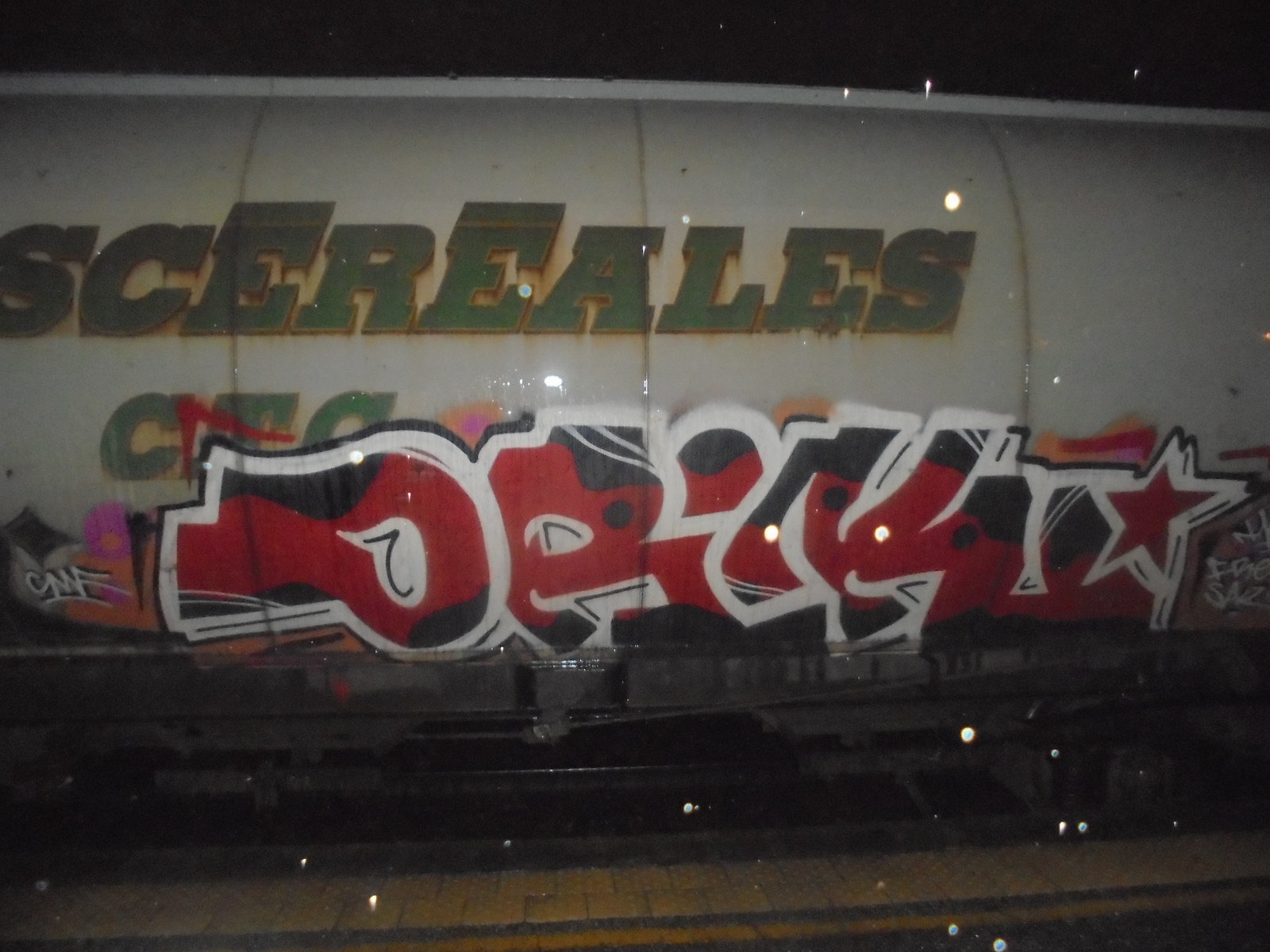The photograph showcases graffiti on a white, cylindrical, train car typically used for transporting liquids or gases. The surface bears green text, "S-C-E-R-E-A-L-E-S C-T-C," which is partially cut off and unclear whether it is part of the graffiti or the train car's labeling. Below this, a series of intricate graffiti patterns dominate the car's lower section, combining red, black, and white colors. The graffiti appears to form obscure shapes and potentially includes a sideways "P," an "R," and the number "44," along with a red star. The scene is set against visible train tracks and a cobblestone or tile floor, suggesting an industrial setting such as a railway yard. The image quality is notably blurred and grainy, adding to the gritty urban atmosphere.